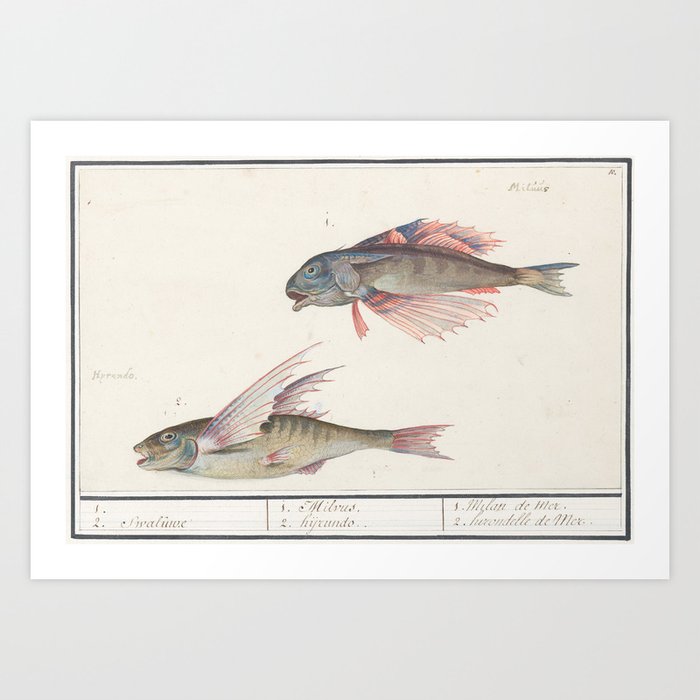This image features a professionally hand-drawn, scientific-style illustration of two fish, each meticulously detailed against a beige background. The scene is enclosed by a thin black line, with an outer white frame, all displayed against a light grayish-blue wall. 

The top fish has a slightly chubbier head with a narrow mouth and blue eyes, adorned with colorful blue-orange-pink fins that resemble bird feathers; its large fin is positioned beneath its body, and its tail extends to the right. It gazes to the left. Below it, the second fish is oblong with notably long, wing-like green fins, a red-tinted tail fin, gills, and a small eye, also looking to the left.

The lower portion of the painting features handwritten descriptions and names for both fish, though the text is mostly illegible. These notes are segmented into three parts, with numerals '1' and '2', indicating some form of identification or classification. Additionally, the illustration is signed by an artist whose name appears to begin with an 'H', and a prominent word starting with 'M' is inscribed at the top of the image.